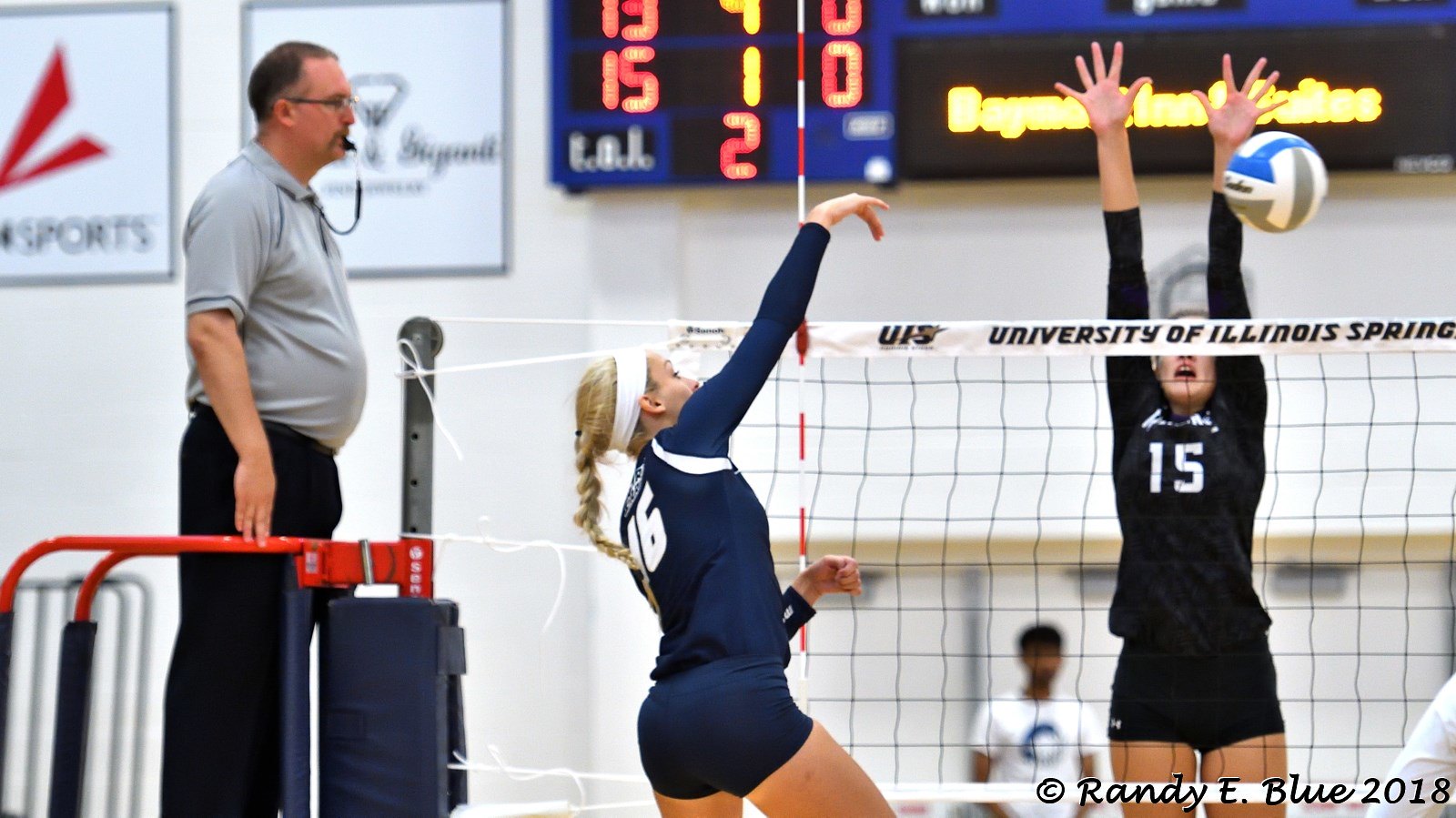This detailed photograph captures an intense moment in an indoor volleyball game, likely taking place in a gymnasium. The image is cropped to prominently feature the top of the net, displaying two players and their mid-air confrontation. 

To the center left, a young, blonde, Caucasian woman with her hair in a ponytail, wearing a white sweatband, dark blue jersey, and dark blue shorts, leaps up at the net. Her jersey reads the number 16 in white on her back, indicating her as a member of one team. She has just hit the volleyball, which is a mix of white, blue, and light gray, now visible at the top right of the image, near her extended right hand.

Opposite her, to the center right and on the other side of the net, stands her opponent—a teenage-looking Caucasian girl in a black jersey and black shorts with the number 15 in white on the front. Her head is obscured by the net, but her outstretched arms and hands are clearly attempting to block the ball, which is just to the right of her extended right hand.

Above the net, the words "University of Illinois Spring" are visible in black text on a white strip. On the top right, a blurry scoreboard, predominantly dark blue and black, adds to the competitive ambiance. 

To the left, a referee intently watches the game, standing on a red-railed podium. This Caucasian man, donning glasses with black frames, has short black hair, wears a tucked-in light gray polo shirt and black slacks, and keeps a whistle in his mouth. Behind him, partially obscured square signs with black text can be found to the left side of the image.

In the distant background, a blurry figure, possibly a coach or spectator in a white t-shirt, stands in front of off-white double doors, adding depth to the scene. The photograph is credited to Randy E. Blue in 2018, marked discreetly in small black text at the bottom right corner.